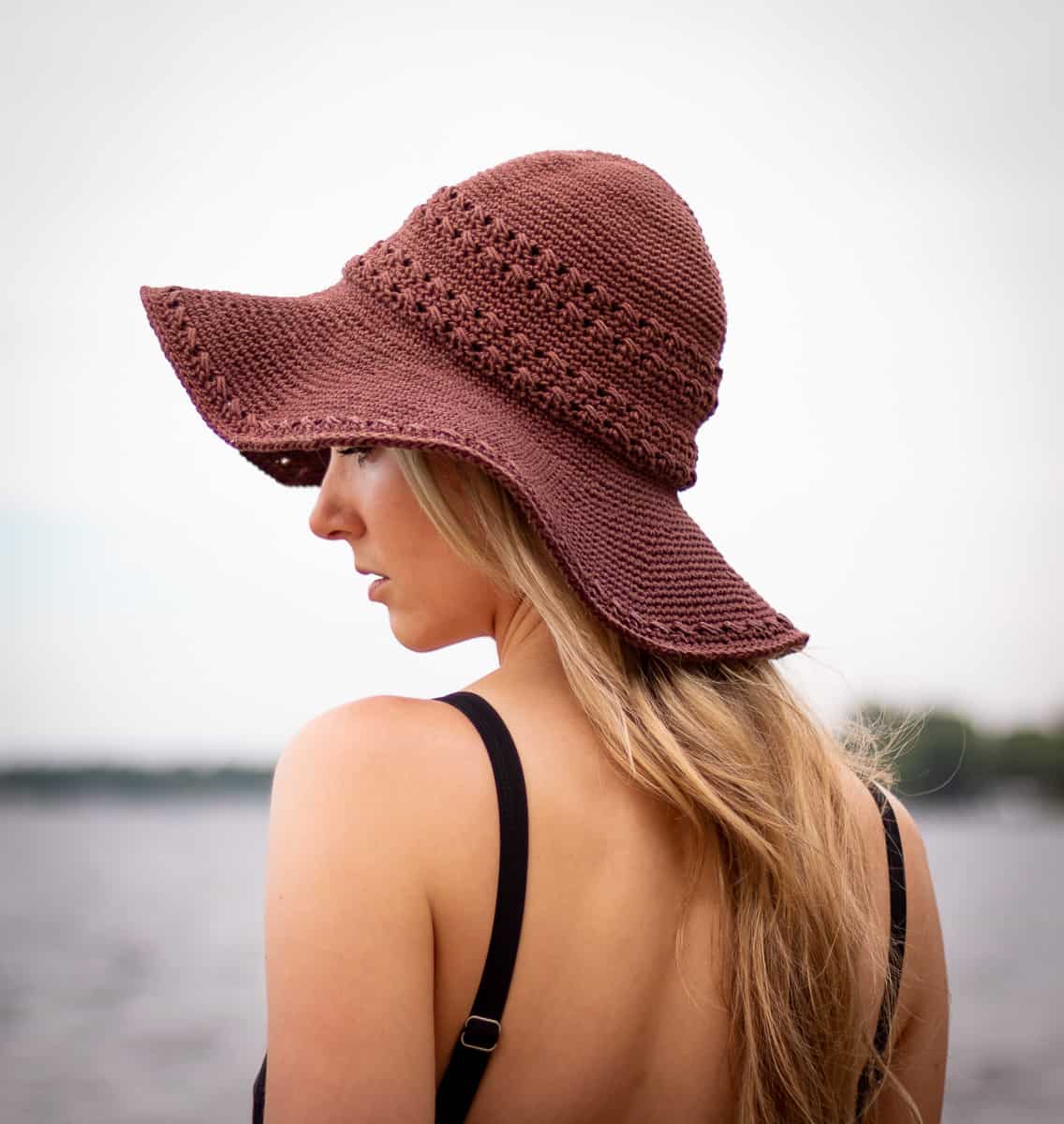This image captures a young woman with long blonde hair, facing a body of water that might be a river or lake, with lush green foliage in the background. Her profile shows her looking slightly down and to the left, standing centrally in a wide vertical frame. The sky appears gray and overcast. She is adorned in a bathing suit with black straps over her shoulders and is wearing a burgundy, intricately woven or crocheted hat featuring two ornate bands and a wide, floppy brim. The focal point includes both her hat and the serene, blurred natural setting, suggesting an outdoor, possibly beachside scene.